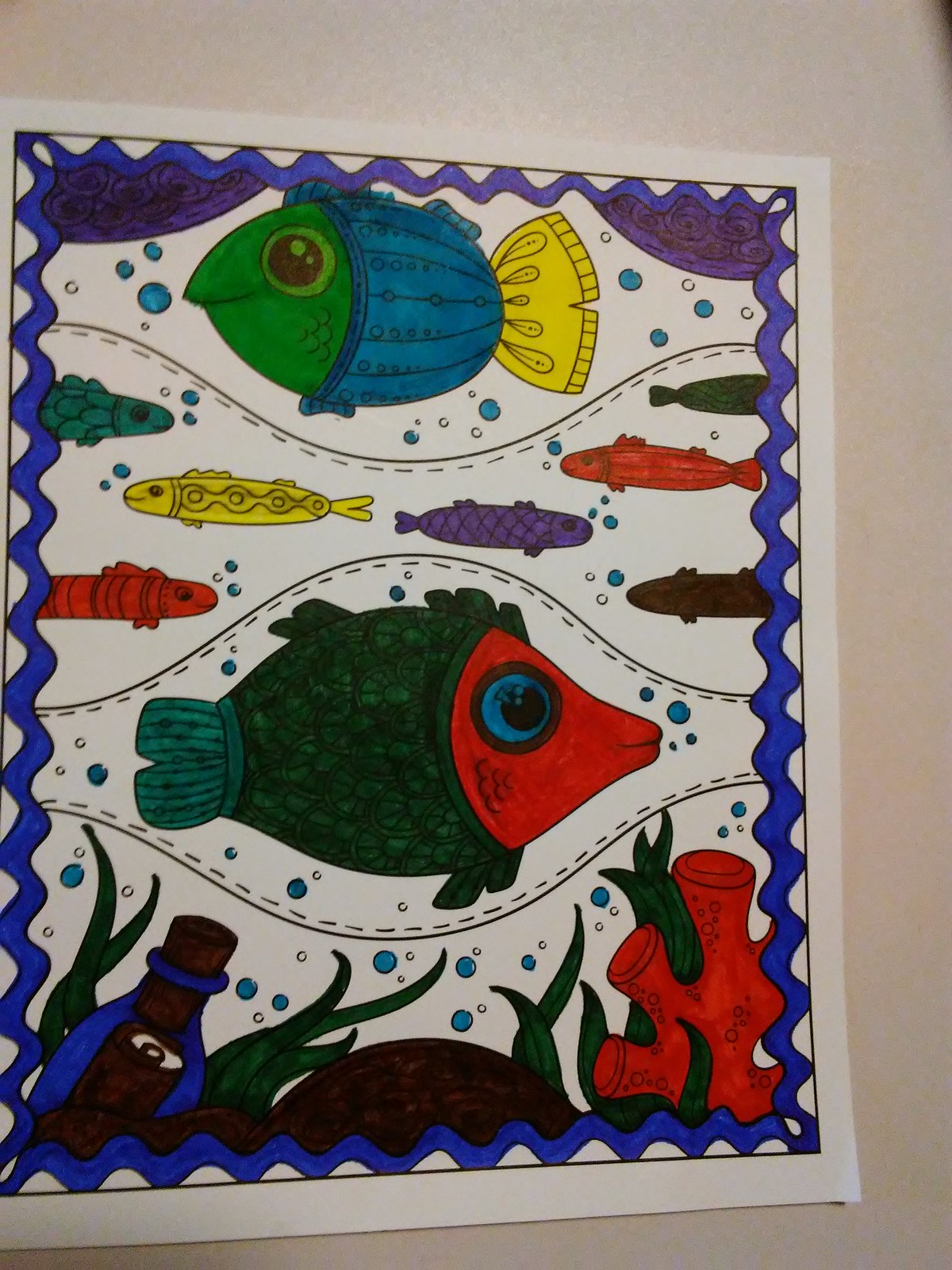On a gray background, a central piece of paper with a white border displays an intricate underwater scene. The scene features two main fish: one positioned at the top left and the other at the bottom right. The bottom right corner has a striking red element. Seaweed is scattered throughout, particularly noticeable on the bottom left side, which also features an eye. The top section of the image is adorned with a range of colors including dark blue waves and a splash of purple on the top right. Amidst this scene, a green fish with a blue body and a yellow tail stands out prominently.

Bubbles are scattered around, with clusters on the left, right, and bottom. Dash marks and lines create a sense of movement. Additionally, several fish populate the scene: a green fish at the top left and middle left, a red fish at the bottom left, another red fish accompanied by a purple fish at the top right, and a purple fish at the bottom right.

In the very center, a distinctive fish with green scales, a red head, and a colorful eye completes this vivid underwater tableau. This fish appears to be in a natural and relaxed state, contributing to the overall harmony of the scene.